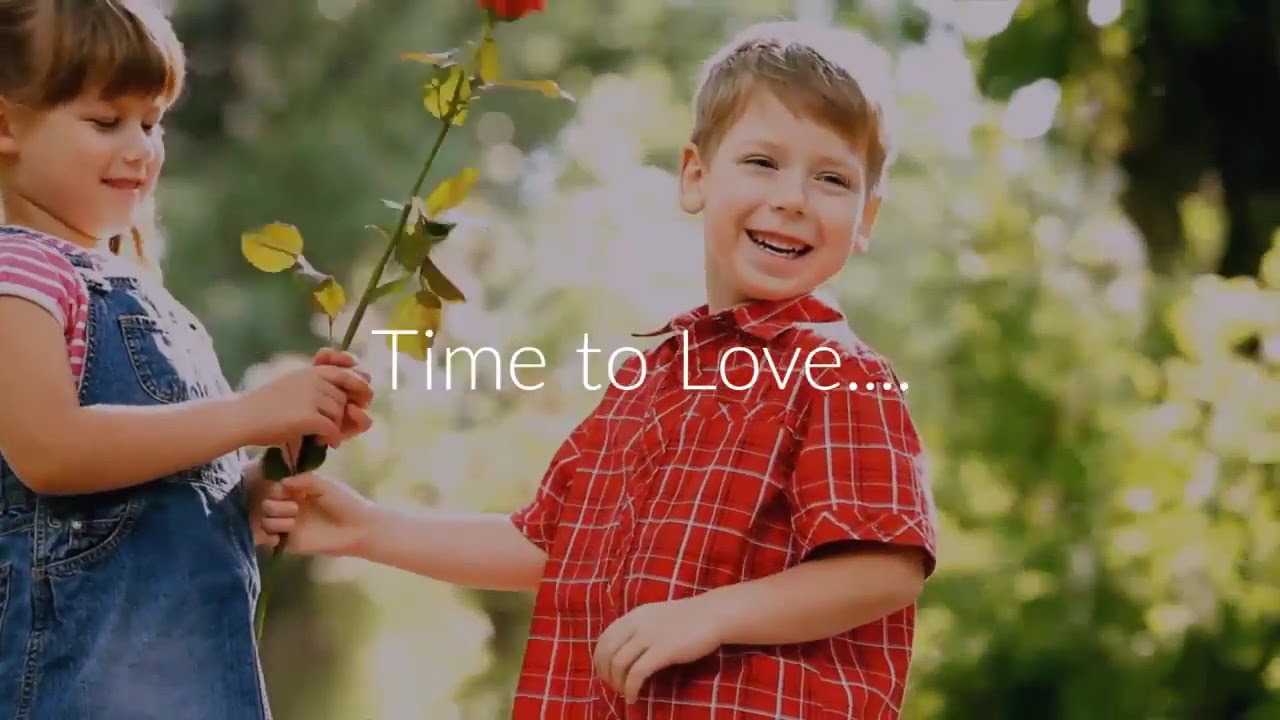The photo captures a tender moment between two Caucasian children, approximately six or seven years old, standing in a forest setting with blurred greenery and trees in the background. Central to the image is a light brown-haired boy wearing a short-sleeved, red collared shirt with white and black stripes. He smiles warmly at the camera as he holds out a green stem with a rose at the top, which he and the girl beside him hold together. The girl, who has brown hair, wears blue jean overalls over a pink and white striped top, and she gazes down at the flower, her hands gently grasping its stem. The scene is overlaid with white text in the middle of the photo that reads, "Time to love...."